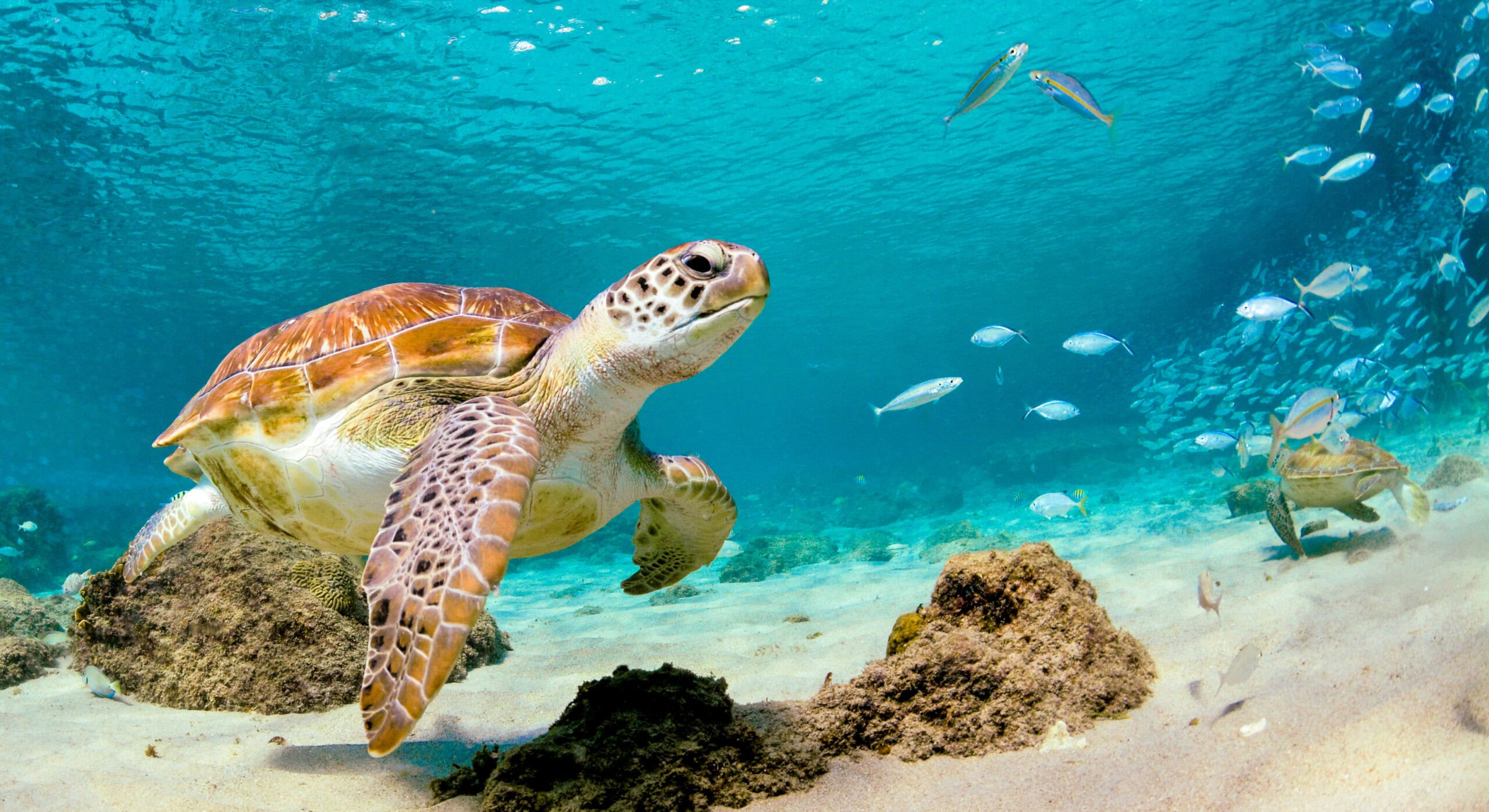This underwater photograph captures a vivid scene in the crystal-clear, true-blue waters of a shallow sea. Dominating the left-hand side is a large turtle with a brown shell and a white underbelly adorned with intricate yellow patterns. Its front fin is primarily brown with striking white square-like markings and some black spots near its eye. The turtle is swimming close to the sandy seabed, which is dotted with brown rocks and possibly some crabs. In the background, on the right side, there's a glimpse of another turtle, partially hidden and distant. To the left near the sand, a baby turtle can be seen. The water above reflects a light aquamarine blue, with sunlight penetrating the shallow depths, illuminating the scene brightly. A school of silver fish swims toward the right, adding to the dynamic marine life captured in this high-definition, vibrant underwater ecosystem.